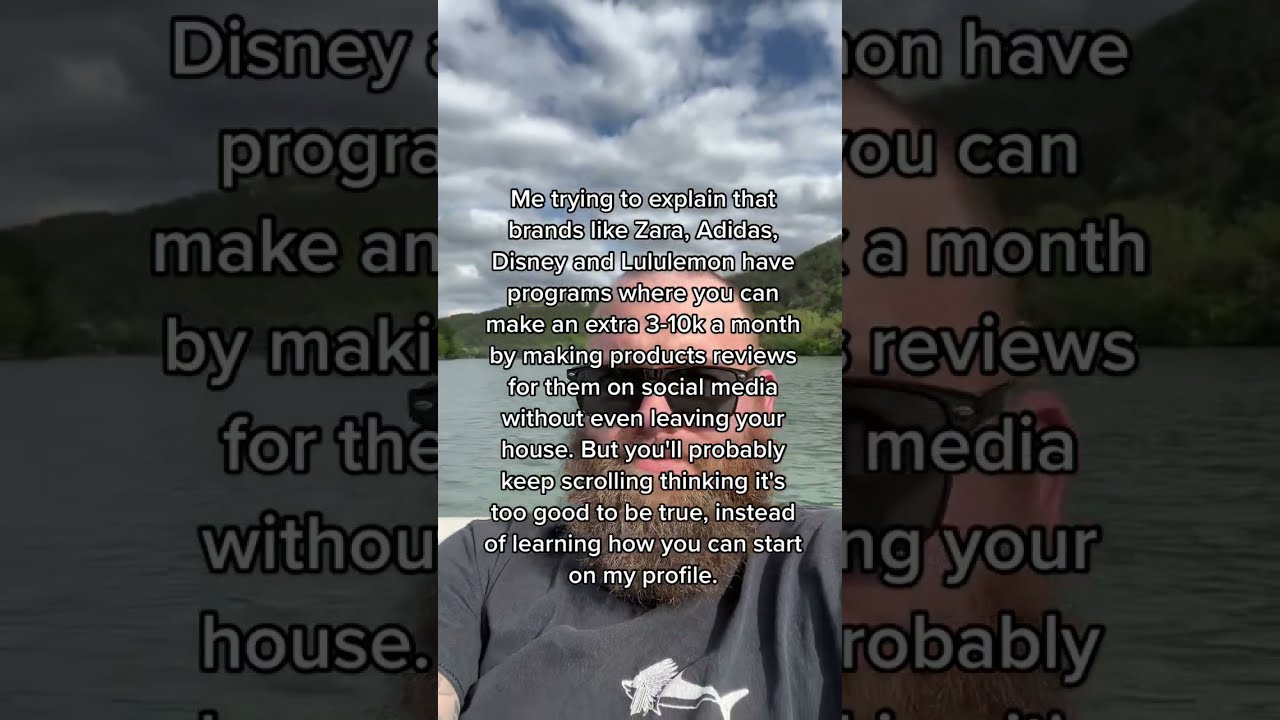The image depicts a man with a bushy brown beard and sunglasses, wearing a dark gray T-shirt with a white fish graphic. He is looking directly at the camera while possibly on a boat, as indicated by the white object in the background. Behind him, there's a scenic view of a body of water, green trees, and a bright blue sky dotted with white clouds. The setting suggests it is daytime. Overlaying the image, centered and in white text, is a caption that reads: "Me trying to explain that brands like Zara, Adidas, Disney, and Lululemon have programs where you can make an extra $3-10k a month by making product reviews for them on social media without even leaving your house, but you'll probably keep scrolling thinking it's too good to be true instead of learning how you can start on my profile." The overall style resembles a screenshot from a TikTok video.